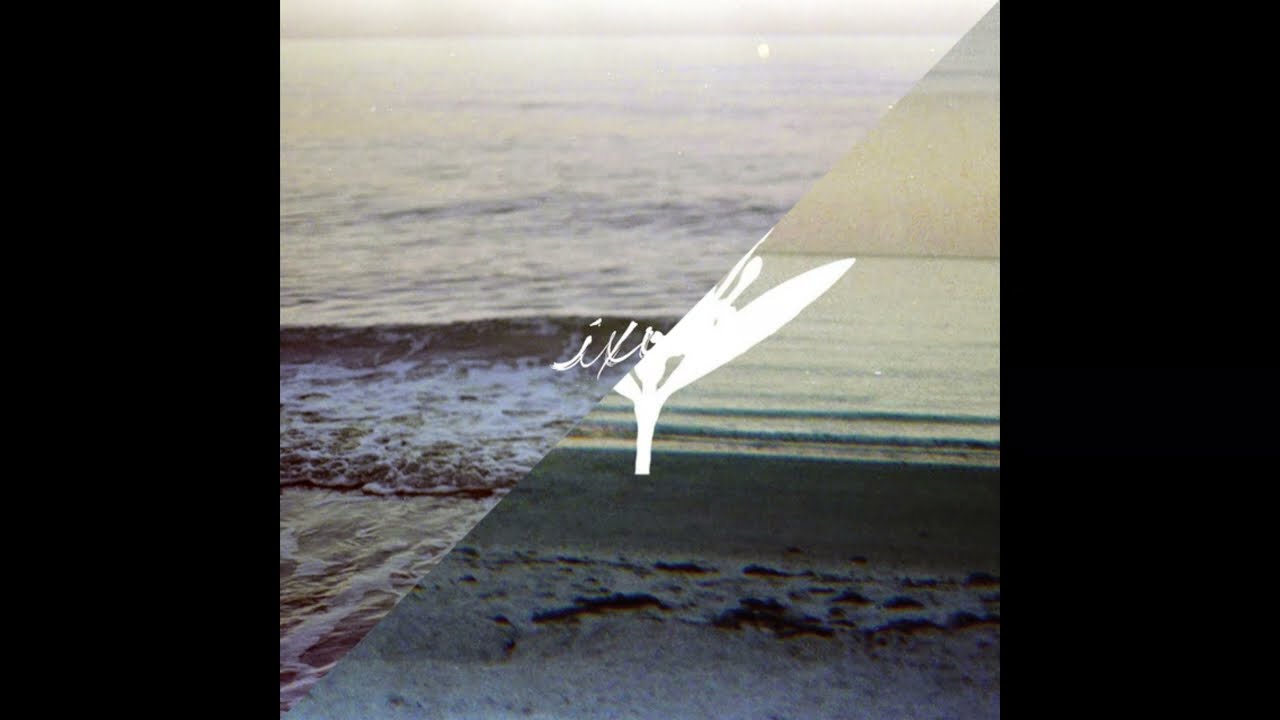The image is a square photograph split diagonally from the bottom left-hand corner to the top right-hand corner, merging two distinct images of beach environments. The left half features a vast ocean with turquoise and dark blue hues, adorned by white cursive letters "IX." The right half, in contrast, showcases a similarly expansive ocean view extending towards the horizon, marked by hazy, mixed colors including orange, and also featuring a prominent white abstract flower in the center with visible petals and stem. Both sides of the image are detailed with visible sandy shores and foamy waves, though the right side is notably grainier with more visible sand and sky, indicating a difference in lighting and texture between the two merged photographs. The entire composite is framed by black rectangles running vertically along the sides.